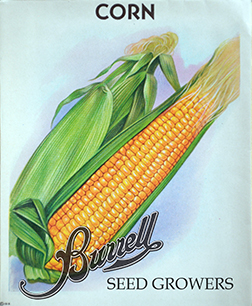The image is an old art piece featuring a highly detailed illustration of two corn cobs. At the top, the text "CORN" is prominently displayed in bold, all-caps lettering. The background transitions from a light blue at the top to a darker blue closer to the corn, adding depth to the composition. In the center, slanted from the bottom left to the top right, are two corn cobs. The corn cob in the foreground has its leaves pulled back, revealing vibrant yellow kernels that stretch along its length, detailed with intricate shading and highlights. Behind it, the second corn cob remains fully wrapped in its green leaves. Beneath the corn, the word "BURRELL" is written in a fancy, cursive font, possibly with a white outline for emphasis, and below that, in thinner letters, are the words "SEED GROWERS." This elaborate illustration appears to be an advertisement for Burrell seed suppliers.